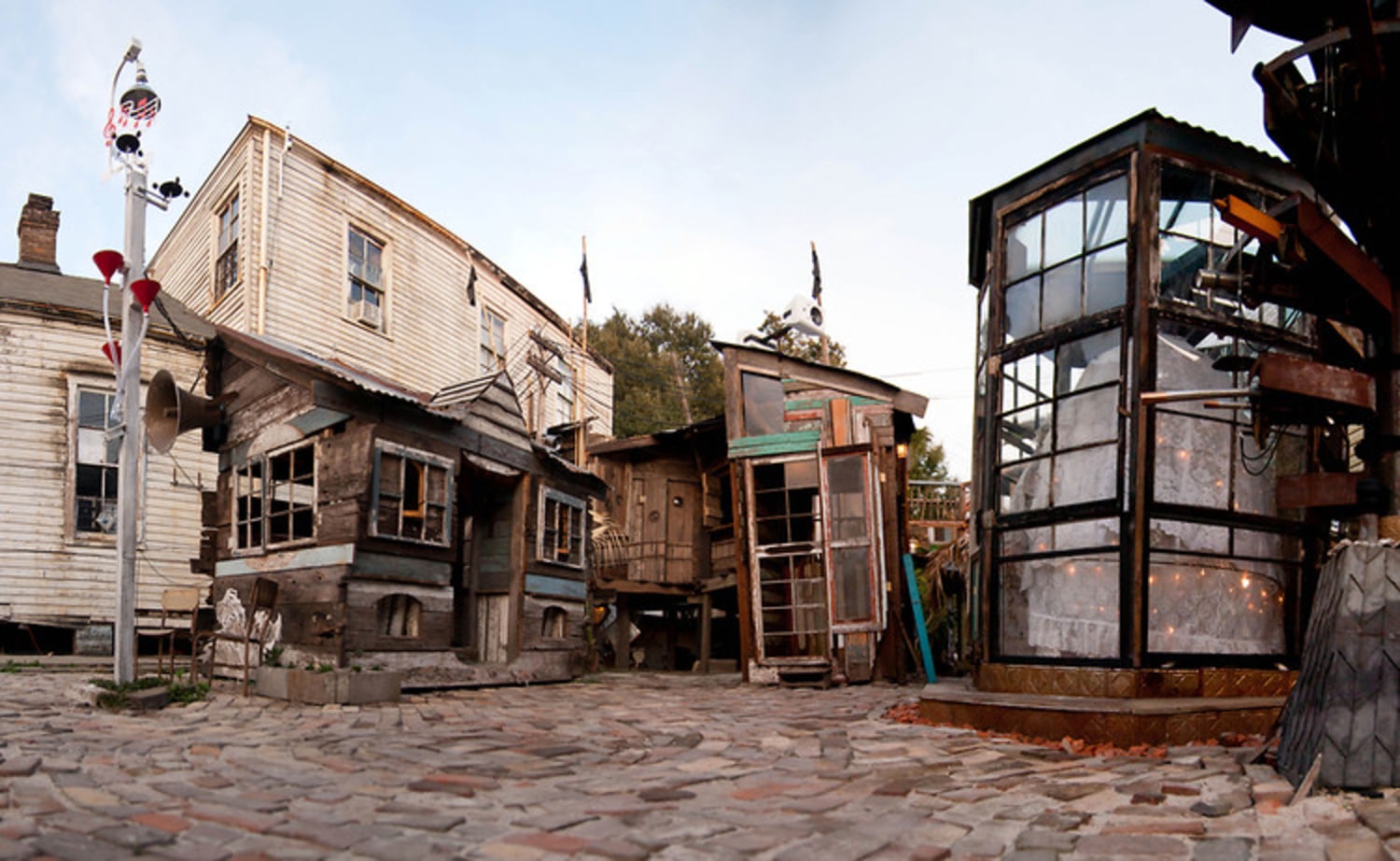The outdoor scene depicted in the color photograph shows a striking display of complete destruction and decay. The ground is composed of unevenly laid cobblestones, creating a rugged, tiled appearance. Under the blue sky, the image features several old, decrepit buildings and structures angled oddly, contributing to a sense of disarray. To the left stands a beige wooden house, which is notably ruined and in dire need of paint. This house is adorned with numerous old windows. Among the other warped buildings is a peculiar one with three small floors framed in wood and featuring glass windows, suggesting an unusual architectural style. Fronted by a tall white pole with painted logos and a megaphone-like structure in red and black, one building further enhances the chaotic atmosphere. Although not immediately identifiable, these structures might be part of an unusual artistic installation or simply remnants of a once lively area now reduced to a state of rustic decay and destruction.